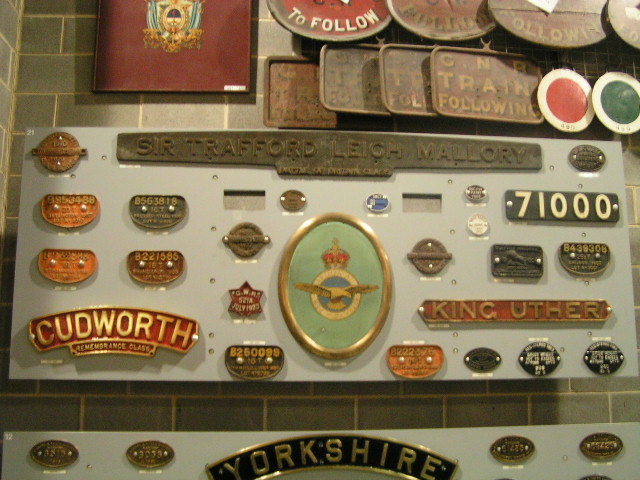This is a detailed color photograph of a display wall adorned with various metal placards, plates, and pins of differing shapes and sizes. The wall itself is made of gray-brick tiles, providing a rustic backdrop. The display comprises at least two primary blue boards set against the bricks. 

On the bottom board, there are several metallic elements including multiple gold oblong placards near an arch-shaped plaque that prominently features the word "Yorkshire" in gold lettering on a black background. Toward the middle, there’s a blue placard inscribed with yellow numbers, and adjacent to it is a bright orange plaque, followed by another oval-shaped and a couple of black plaques. The name "Cudworth" is also visible on the lower section. Centrally placed amongst the plaques is a design resembling a clock with a crown on a green background. The right side of the same board features the name "King Uther" along with the number "71000".

The top board also showcases an array of plaques and pins, with one prominently featuring "Sir Trafford Leigh-Mallory" across the top. Among these, there is a plate labeled "CNR train following" and several round and square metallic symbols, possibly old license plates or train-related memorabilia. Each element of this collection appears intricately designed, indicating it might belong to a collector of vintage and railway memorabilia.